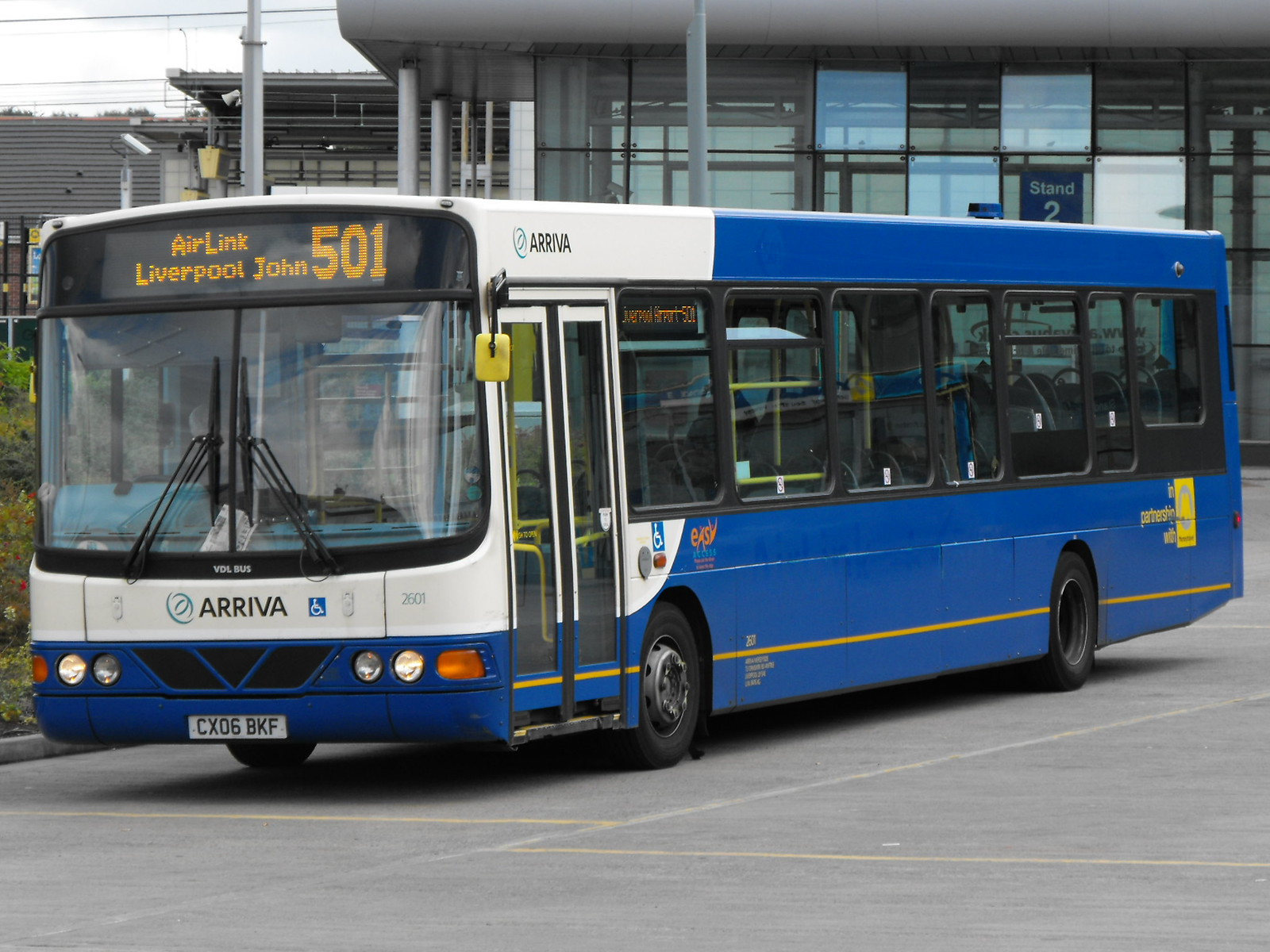The image captures a large, royal blue and white single-decker bus parked in the parking lot of a bus stop on a cloudy day. The bus, identifiable as an Arriva bus, bears the text "Airlink Liverpool John 501" in orange on a screen at the front. Its body is mainly blue with yellow stripes running along the bottom and a white front section where "Arriva" is painted in black alongside a square with a disabled icon. The license plate reads CX0XBKF. The bus is photographed from an angled view, displaying both its front and left side, with clear, curved glass windows fitted with windscreen wipers. Four lights are located at the front, with additional orange lights on the outer edges. The bus features two double doors on the front side and numerous windows lining its length. It is positioned in front of a bus depot or large glass building with a visible white awning, and some solar panels can be seen in the background. The area around the bus is devoid of people.